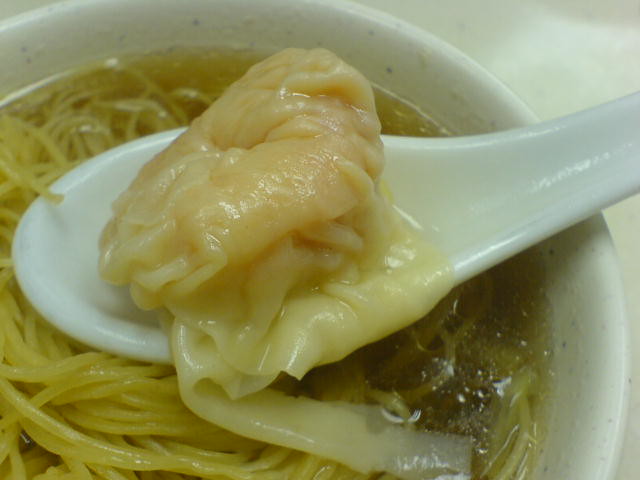This color photograph, oriented in landscape, captures a white glass or ceramic bowl filled with a mix of thin, soup-like noodles submerged in a clear, yellow-brown broth. A prominent white porcelain spoon, resting horizontally across the bowl from the right to the left side, holds a large, semi-translucent dumpling that appears wet, suggesting it has been steeped in the broth. The dumpling or possibly a piece of meat, has a similar coloration to the noodles, making it appear somewhat ambiguous. The scene is set against a white tablecloth, enhancing the bowl's pristine appearance and emphasizing the detailed realism of the food.